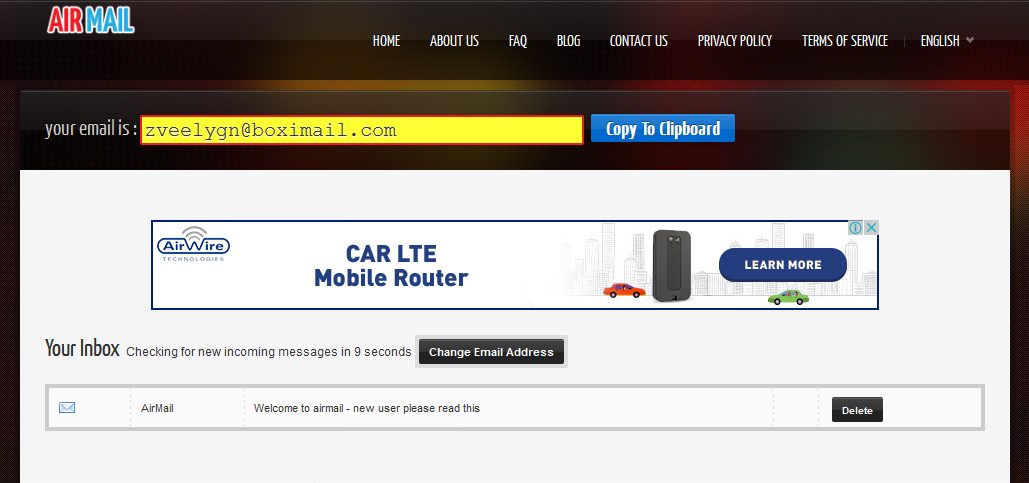This is a detailed screenshot from the Airmail website. The top section features a dark brown background with the Airmail logo on the left: "AIR" in bold red with a white outline and in all caps, followed by "MAIL" in light blue, also in all caps with a white outline, making up "AIRMAIL." 

To the right of the logo, there are several navigation tabs in white text on the brown background: HOME, ABOUT US, FAQ, BLOG, CONTACT US, PRIVACY POLICY, TERMS OF SERVICE, and a drop-down menu for language selection labeled ENGLISH.

Beneath the header, the background shifts to an orangey-yellow-brown hue. The foreground displays a centrally positioned brown box. Inside this box, white text reads "YOUR EMAIL IS," followed by a yellow box with a red outline containing the email address "ZVELLIGN@BoxEmail.com" in black text. Below this, a medium blue tab labeled "COPY TO CLIPBOARD" in white text allows users to copy the email address.

Lower on the page, there is an advertisement for a "CAR LTE MOBILE ROUTER" from AIRWIRE. Directly beneath this ad, a white box with black text states, "YOUR INBOX CHECKING FOR NEW INCOMING MESSAGES IN 9 SECONDS," with an option to change the email address.

Finally, the inbox section contains a welcome message titled "WELCOME TO AIRMAIL," with a subheading for new users: "NEW USER PLEASE READ THIS." There is also an option to delete this welcome email.